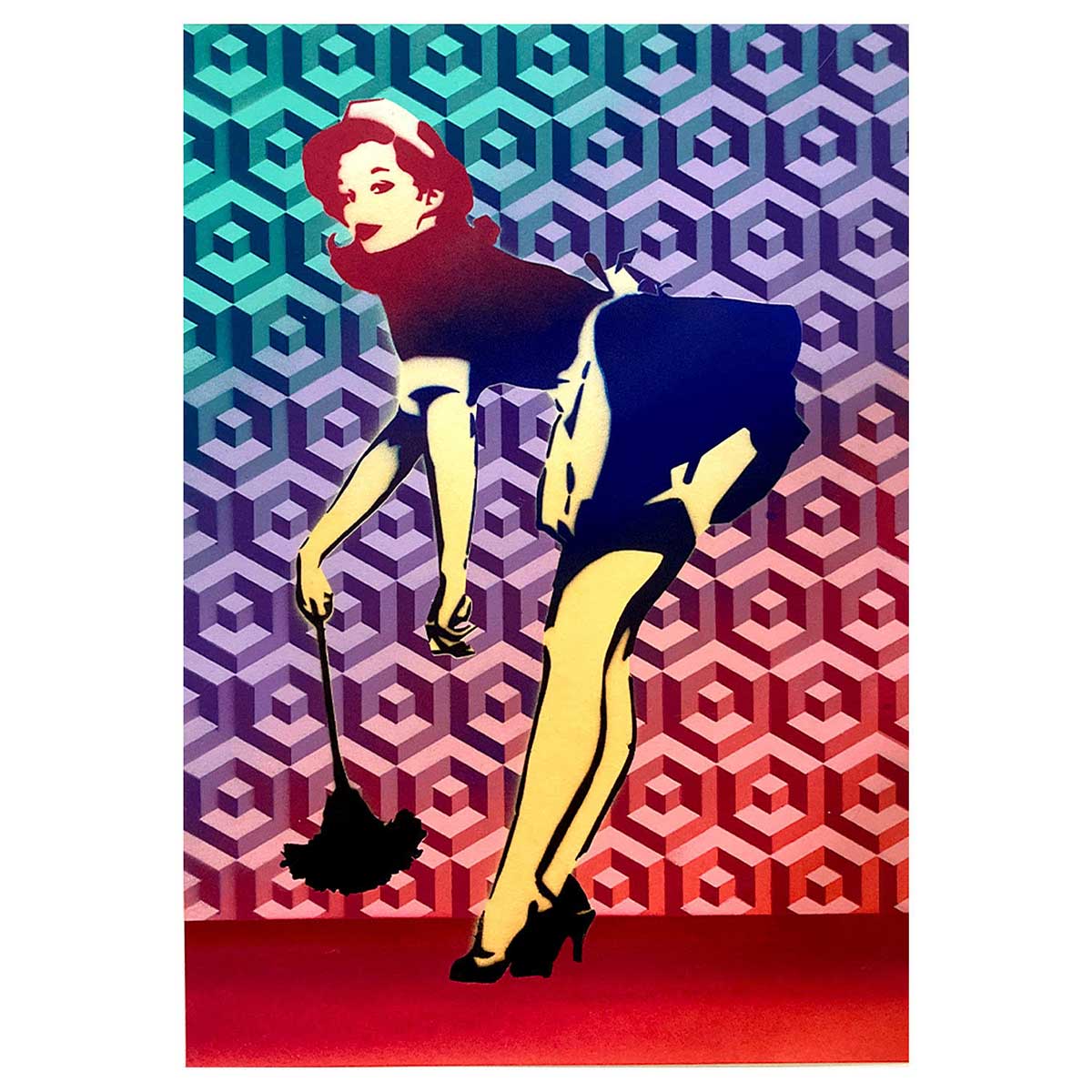This illustration is a vibrant and modern pop art stencil depicting a pin-up style maid bent over provocatively at the waist, facing to the left. She sports a traditional maid costume with a white cap atop her brunette hair, red lips, and black high heels. Her attire includes a navy blue short-sleeved shirt trimmed in white, a very short navy blue skirt, a white apron, and thigh-high stockings with visible garters. In her right hand, she holds a black feather duster pointing towards the ground.

The background showcases a striking geometric array of 3D cubes in a vivid color gradient moving diagonally from top left to bottom right, transitioning from teal blue, to light purple, followed by dark red. The floor beneath her is similarly dark red, complementing the color palette. The maid’s skin tone is a yellowish-pale, adding to the modern pop art aesthetic of the piece.